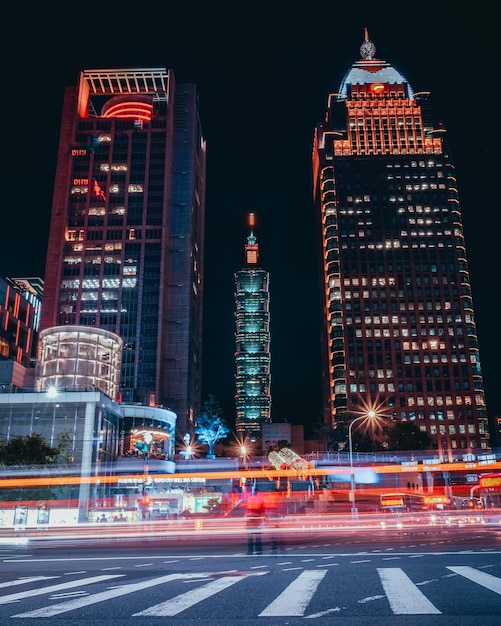Captured at street level, this vibrant nighttime cityscape showcases a bustling intersection illuminated by dynamic streaks of light, likely the result of a long exposure capturing the movement of speeding traffic. Framing the scene are three prominently featured buildings. On the right stands the widest structure, approximately 25-30 stories tall, adorned with numerous smaller windows and crowned with a blue tip and a glowing globe, bathed in orange light. To its left is a similarly tall but more modern building with larger windows. The building in the middle, further in the background, appears slightly shorter and is illuminated in blue and green lights with a blue and orange tip. At street level, a glass circular building is visible at the base of the left structure, alongside streetlights flashing pink and a tree lit with green lights. The entire scene exudes the energetic ambiance of a busy city intersection.